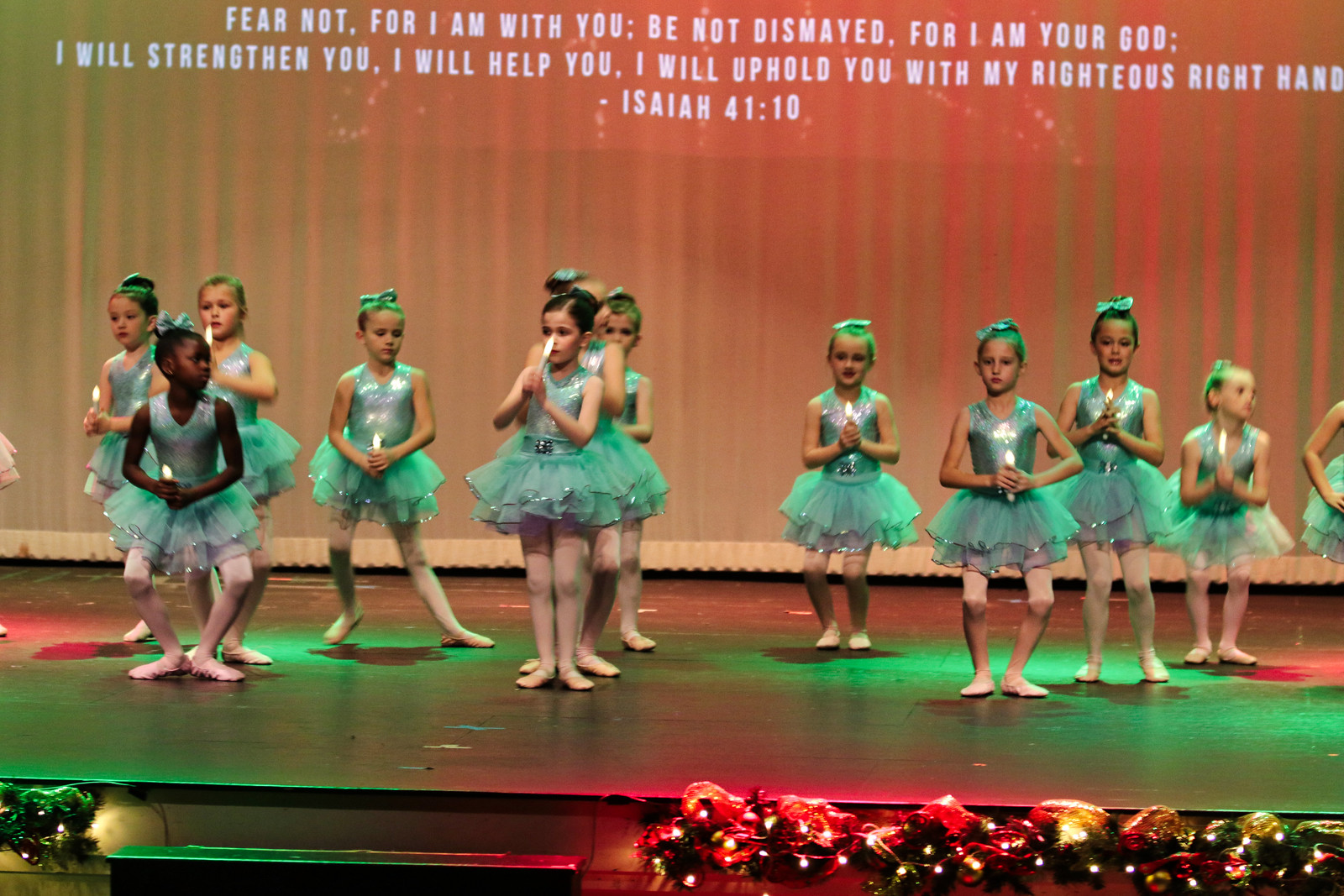The image captures a group of young girls on a stage, all dressed uniformly in blue ballerina outfits, consisting of sleeveless tops, sheer blue tutus, and white tights. The black stage is framed with white-painted wooden steps leading up to it, and festively decorated with green garlands intertwined with various colored Christmas tree lights, adding to a holiday atmosphere. Above the stage, a white curtain wall serves as a backdrop, with a Bible verse from Isaiah 41:10 projected in white text that reads, "Fear not, for I am with you. Be not dismayed, for I am your God. I will strengthen you, I will help you, I will uphold you with my righteous right hand." The girls appear to be holding battery-operated candles, suggesting a Christmas concert theme, enhanced by the red and green lighting that bathes the stage in a festive glow.